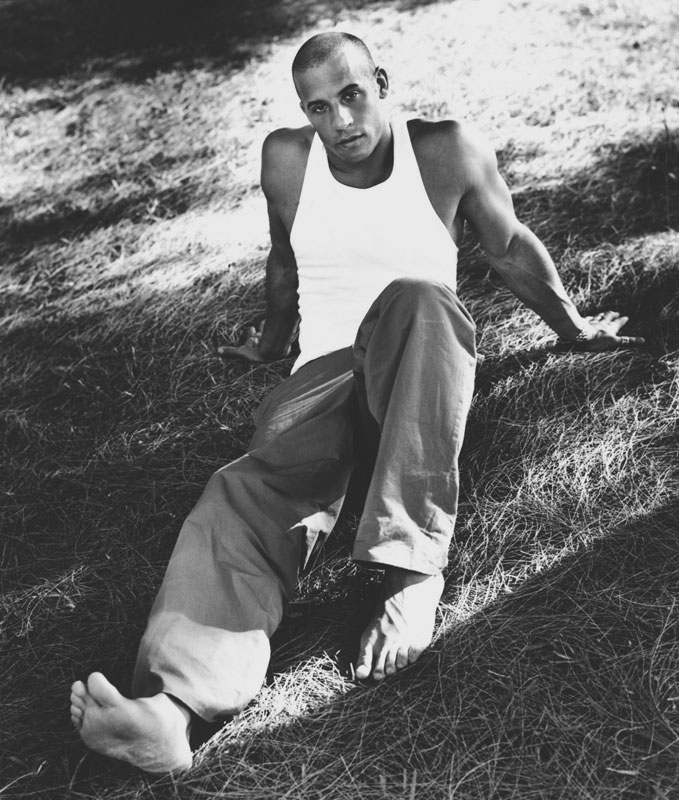This is a striking black and white photograph of a younger Vin Diesel, taken on a sunny day outdoors. In the image, Vin Diesel is sitting on a grassy hillside in the shade, leaning back with his arms supporting his body. His legs are stretched out in front of him, revealing that he is barefoot, with the bottom of his right foot and the top of his left foot visible. He dons a white tank top and loose-fitting long pants, possibly jeans, though the grayscale nature of the photo makes it difficult to determine their actual color. Notably, Vin Diesel has a short military buzz cut, differing from his usual bald look. The natural lighting creates a chiaroscuro effect, enhancing the contrasts and giving the image a highly saturated appearance. Vin Diesel completes his casual look with a watch and ring on his left hand. The photo captures a serene and candid moment of the movie star.